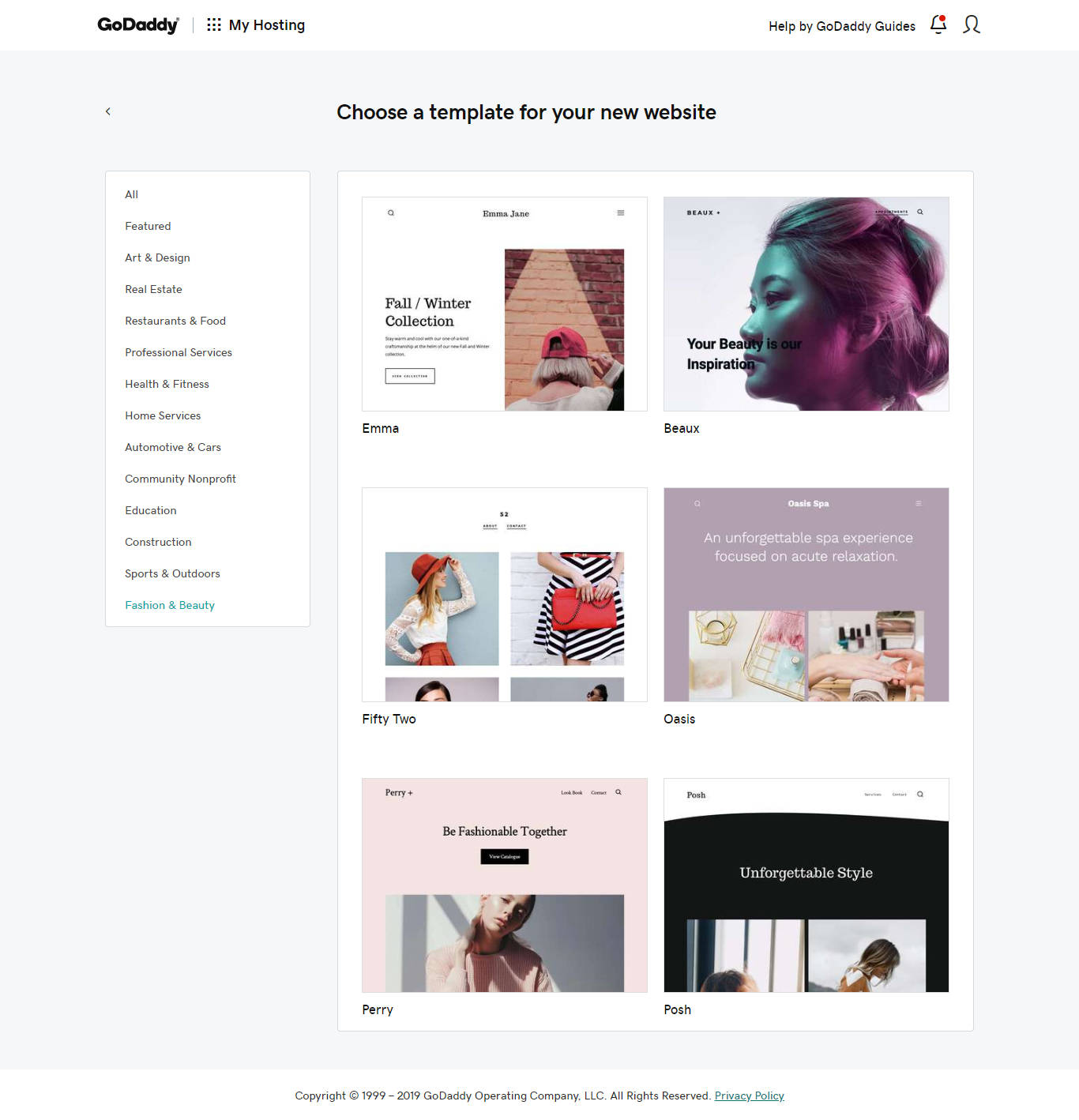The image is a digital interface from GoDaddy's website builder, featuring a user-friendly layout for creating a new website. The main section displays a grid layout of nine squares, arranged in three rows and three columns, resembling a matrix of dots. The interface is branded with "My Hosting Help by GoDaddy Gods" prominently at the top. 

In the upper right corner, there are notification and profile icons. Below, a prompt encourages the user to "Choose a template for your new website." 

On the left side, a vertical navigation panel lists various categories, starting with "All" and ending with "Fashion and Security," which is highlighted in blue, indicating it is currently selected while the rest of the categories are in black text.

The main content area displays a series of image blocks or template previews. The first block showcases a "Fall/Winter Collection" with the word "Emma" beneath it. The second block features the text "Your Beauty" and "Inspiration," with "Beaux" (B-E-A-U-X) written below. 

The third block is a collage of four smaller images: the upper two images show women modeling different outfits, one in a dress and the other in a blouse, skirt, and hat, with the number "52" displayed adjacent. The bottom two images are cropped to feature parts of two women's faces.

Another series of blocks includes an image emphasizing makeup products labeled "Oasis" and another with the text "Perry."